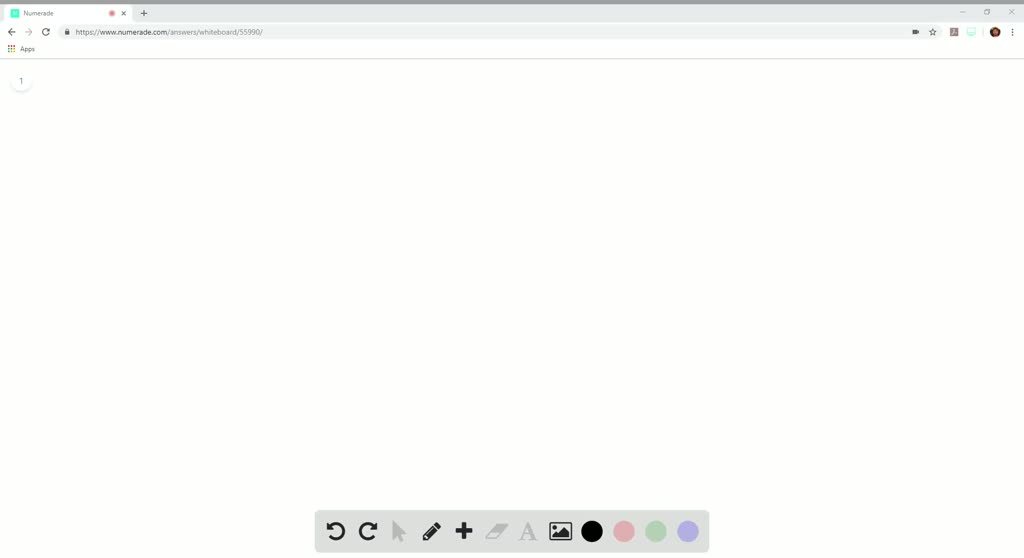The screenshot captures a predominantly white web page with a header and navigation bar. The top-left corner displays a blurry browser tab labeled "NumerAid" alongside a light green square icon. Just beneath is the address bar, showing the URL "http://www.numeraid.com." Below this bar, there is an "Apps" icon with the word "apps" in dark gray text next to navigation arrows and an undo button.

In the upper right corner of the image, set against a light gray header, there is a close window "X" icon. Adjacent to this, there's an icon featuring a black circle containing an indiscernible symbol and a gray square.

The lower section of the web page is highlighted by a lavender box housing several interactive elements: an undo button, a crayon icon, an image button, and four circular color options arranged from left to right—black, pink, light green, and blue. The overall layout and elements suggest a user-friendly interface aimed at providing various interactive tools.